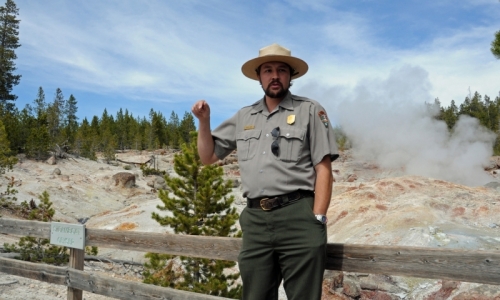The photograph features a park ranger with a tanned complexion and a dark brown or black beard. He is wearing a standard ranger outfit consisting of a wide-brimmed brown hat, a greyish-green button-up shirt with a badge, and dark green pants. He is standing against a weathered wooden fence, which has a sign, although the text on it is illegible. Behind him, the scenery, which looks like it could be from Yellowstone National Park, includes a mix of rocky ground and white and brown fields with noticeable steam venting from the ground. This steam hints at geothermal activity, possibly hot springs, in the area. In the distance, there is a line of pine trees and other types of trees, set against a backdrop of blue sky with wispy clouds.